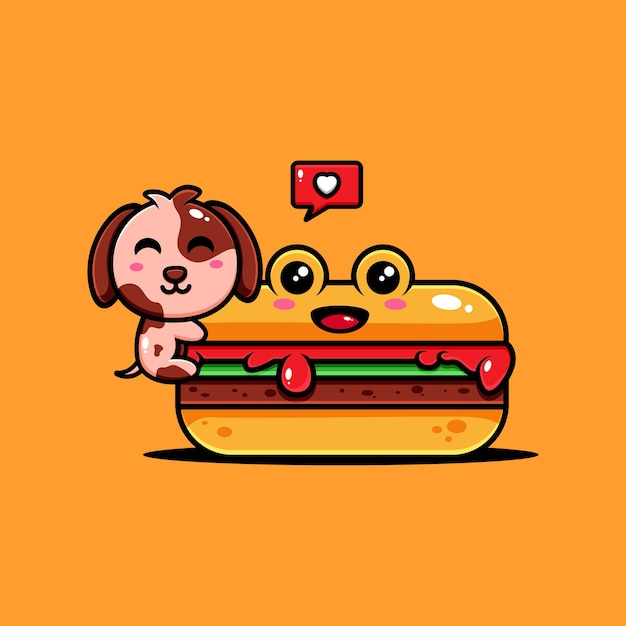This vibrant, digitally illustrated image captures a whimsical, juvenile comic scene set against a solid orange background. Dominating the center is a personified cheeseburger with expressive, wide-open eyes, each featuring black centers and tiny white accents, and a mouth formed with a black outline and a red interior dotted with white. The cheeseburger, constructed with a beige bun speckled with orange dots, showcases layers of ketchup, lettuce, and a beef patty. Beneath its upper bun, pink blush spots accentuate its cartoonish charm.

To the left, a playful pink and brown dog is humping the burger, depicted in a mischievous pose with its profile turned towards the viewer. The dog’s design includes closed eyes, a big smile, prominent pink cheeks, floppy ears, and distinct spots of peach and brown on its body. The dog's raised tail and white spot on its back add to its endearing appearance. Floating above its head is a red speech bubble containing a white heart, indicating its affectionate mood. The overall style of the artwork is reminiscent of nostalgic 80s and early 90s video game graphics.